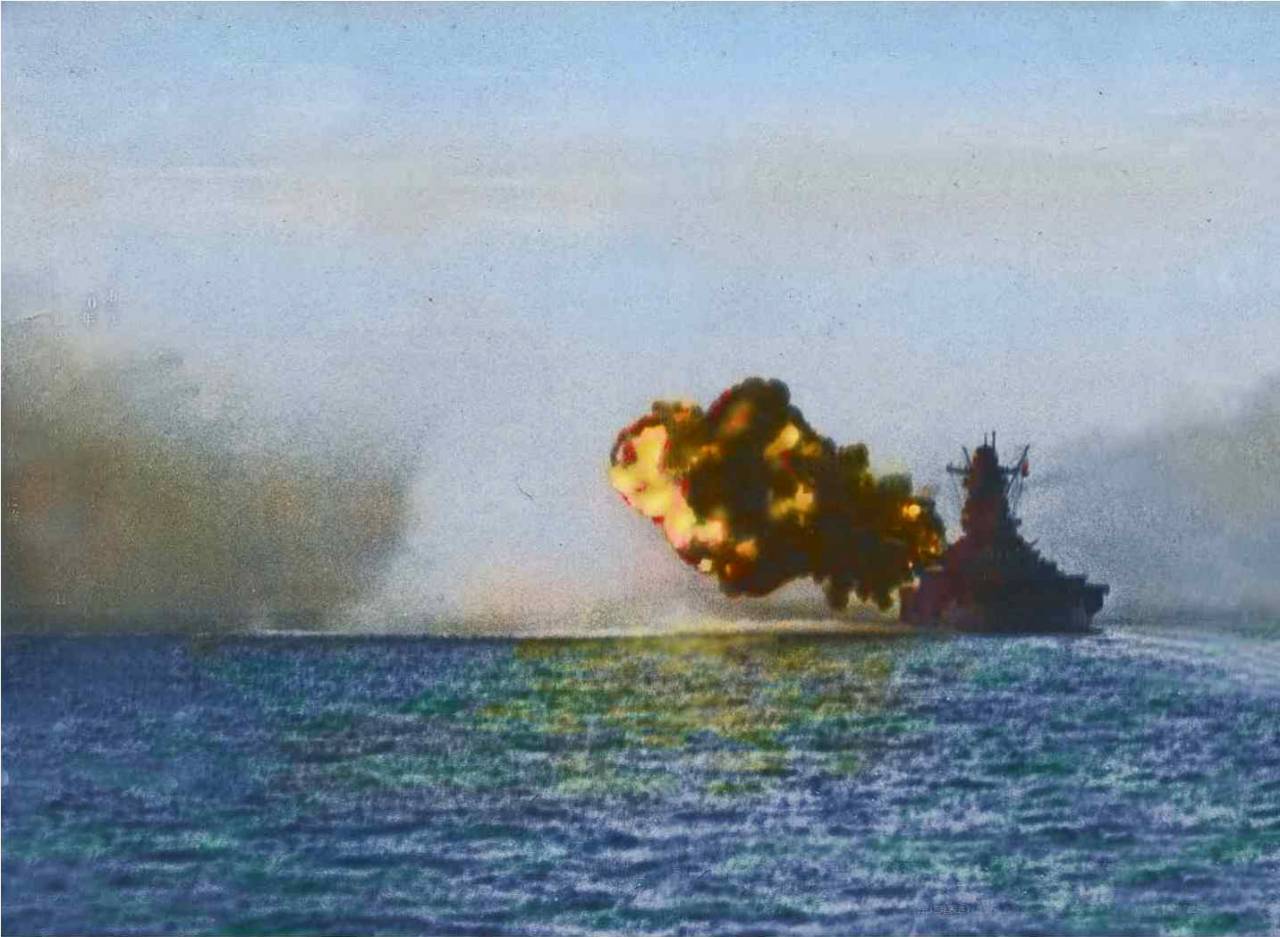In this rectangular, grainy photograph, which appears to have been colorized from an original black-and-white image, an alarming scene unfolds on the open ocean. The focal point is a large warship or vessel positioned on the right side of the image, engulfed in a significant explosion on its left side. Large red, yellow, and orange flames burst violently, accompanied by thick black smoke that billows into the sky. The smoke is interspersed with grayish clouds from previous firings. The ocean water, a mix of bluish-green hues, transitions to a yellowish tinge surrounding the explosion, reflecting the intensity of the fire. The vibrant blue sky contrasts with the dark, heavy clouds lingering on the horizon, creating a dramatic backdrop. The photograph's graininess and artificial coloration suggest it documents a historical event, possibly a wartime scene, underscoring the chaotic and perilous circumstances of the moment.